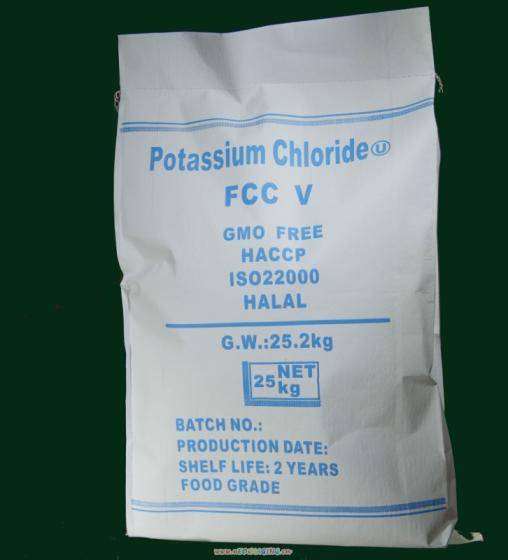This image presents a large white bag with light blue lettering, set against a forest green background. The top of the bag features a drawstring closure. Centered at the top of the bag, the text reads "POTASSIUM CHLORIDE" followed by "FCCV," "GMO FREE," "HACCP," "ISO 22000," and "HALAL." Below this, there is a line of text that includes "GW: 25.2 kg" and a blue box with the weight "25 NET KG." Further down, the text continues with "BATCH NUMBER," "PRODUCTION DATE," and "SHELF LIFE: TWO YEARS." At the bottom of the bag, "FOOD GRADE" is prominently displayed with two thin blue stripes beneath it. The background outside the bag features more unreadable small white print. All the text, except for "POTASSIUM CHLORIDE," is written in capital letters.